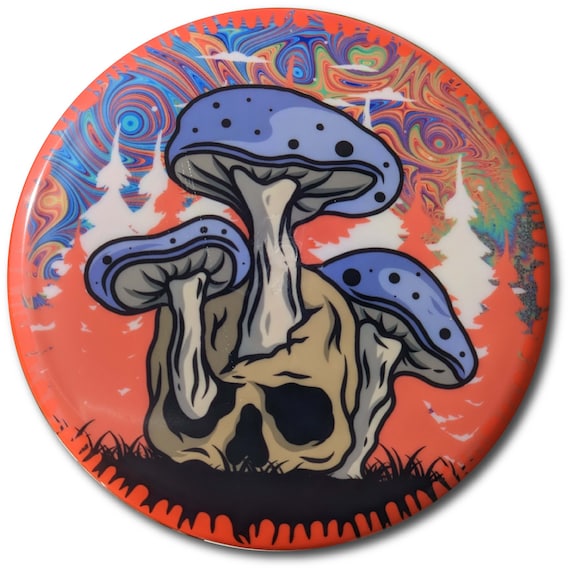The image is a detailed, close-up shot of a circular pin, designed with a myriad of trippy, psychedelic elements reminiscent of the 60s and 70s. The pin's background features a vibrant blend of red-orange, with swirls and circles in blue, green, purple, and yellow, creating an acid-like, LSD-inspired ambiance. Tiny white speckles dot the backdrop, setting a cosmic or starry atmosphere. Amidst this colorful chaos, white and orange outlines of trees emerge.

Central to the design is a large, tan skull, seemingly crafted from clay or earth, resting on a patch of black grass. Three mushrooms sprout from this skull: one from the left eye socket, another from a hole at the top, and the third extends behind. These mushrooms have grayish stems, dark gray undersides, and caps colored in a purple-lilac hue with black spots and holes, adding to the surreal, otherworldly feel of the pin. The image lacks any text, allowing the bizarre and captivating visual elements to dominate.